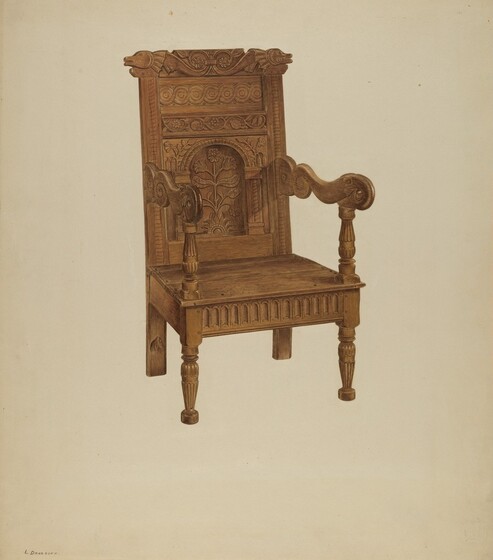The image features a meticulously detailed wooden chair, set against a plain whitish-gray background, giving prominence to the intricacies of the chair itself. The chair boasts high armrests that curve elegantly, leading down to ornately carved front legs that taper into circular knobs at the bottom, embellished with decorative features. In contrast, the back legs are simpler, straight rectangular shapes. The chair's flat wooden seat and back are adorned with intricate engravings, including swirling patterns and floral designs. Notably, the backrest features a carved circular area with a flower design and is topped with an elaborate motif that appears to depict a two-headed animal, possibly snakes or fish. The entire piece exudes an old-fashioned charm, combining both practical structure and artistic craftsmanship, making it clear why it might have been chosen as a subject for this picture.